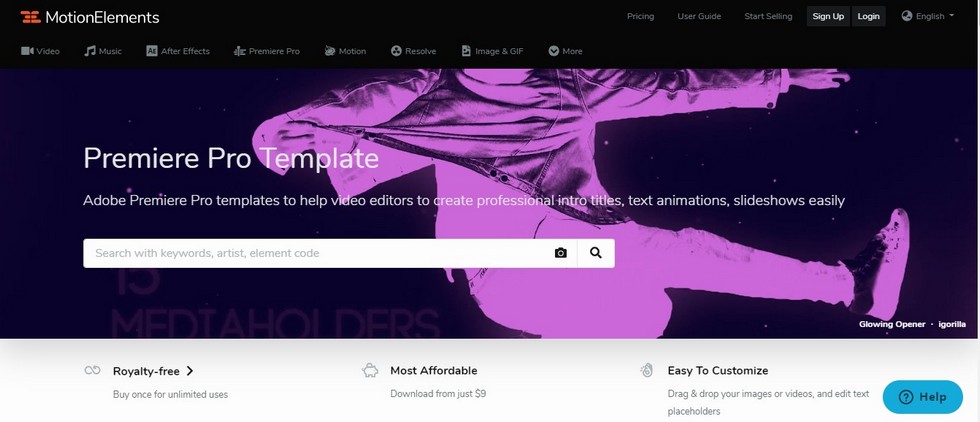The webpage displayed in the image centers around video editing and prominently features a service named "Motion Elements." The top left corner showcases the website name in white text, next to an orange-colored logo consisting of six oval shapes. Adjacent to the left are user interaction options, including "Start Setting," "User Guide," and "Pricing." The top right contains language selection, login, and sign-up buttons presented in separate boxes.

In the middle of the webpage, a visually striking background image of a dancer is tinted light purple, emphasizing the site’s creative focus. Overlaid on the background, the phrase "Premiere Pro Template" is situated on the left, followed by a detailed description: "Adobe Premiere Pro Template to help video editors create professional intro titles, text animations, slideshows easily."

Further down on the left, there is a search box labeled "Search with Keywords Artist Element Code," accompanied by a magnifying glass icon and a camera icon to its right.

At the bottom right of the image, the words "iGorilla" are visible, positioned next to the title "Glowing Opener," separated by a dot, likely indicating the name of a specific project or feature.